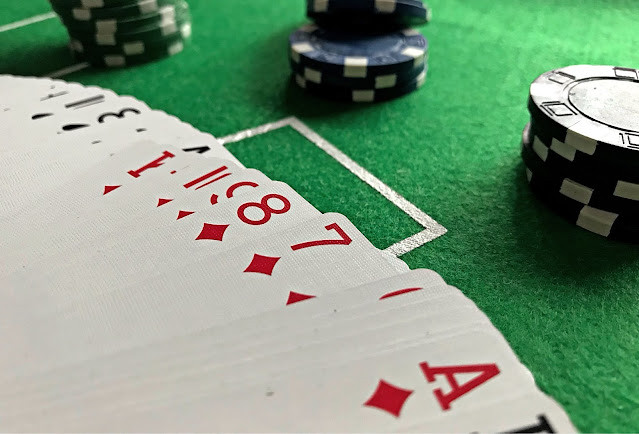This photograph captures a close-up view of a tabletop, either in a casino or a home setting, covered with green felt and marked with white painted squares, only partially visible due to various items arranged on the table. Three orderly stacks of blue and white poker chips are positioned on the green surface: one in the upper right corner, another in the top center, and the last slightly lower to the left. Spread across the table is a deck of playing cards, fanned out to reveal portions of several cards. Prominently displayed in the center are the 7 of diamonds and the 8 of diamonds, overlapping what appears to be the 9 and 10 of diamonds. Towards the lower right, the ace of diamonds is clearly visible with a black jack card partially covering it, leaving the suit undetermined. In the upper left corner, a glimpse of the 3 of spades can be seen, completing this intricate and engaging scene on the tabletop.